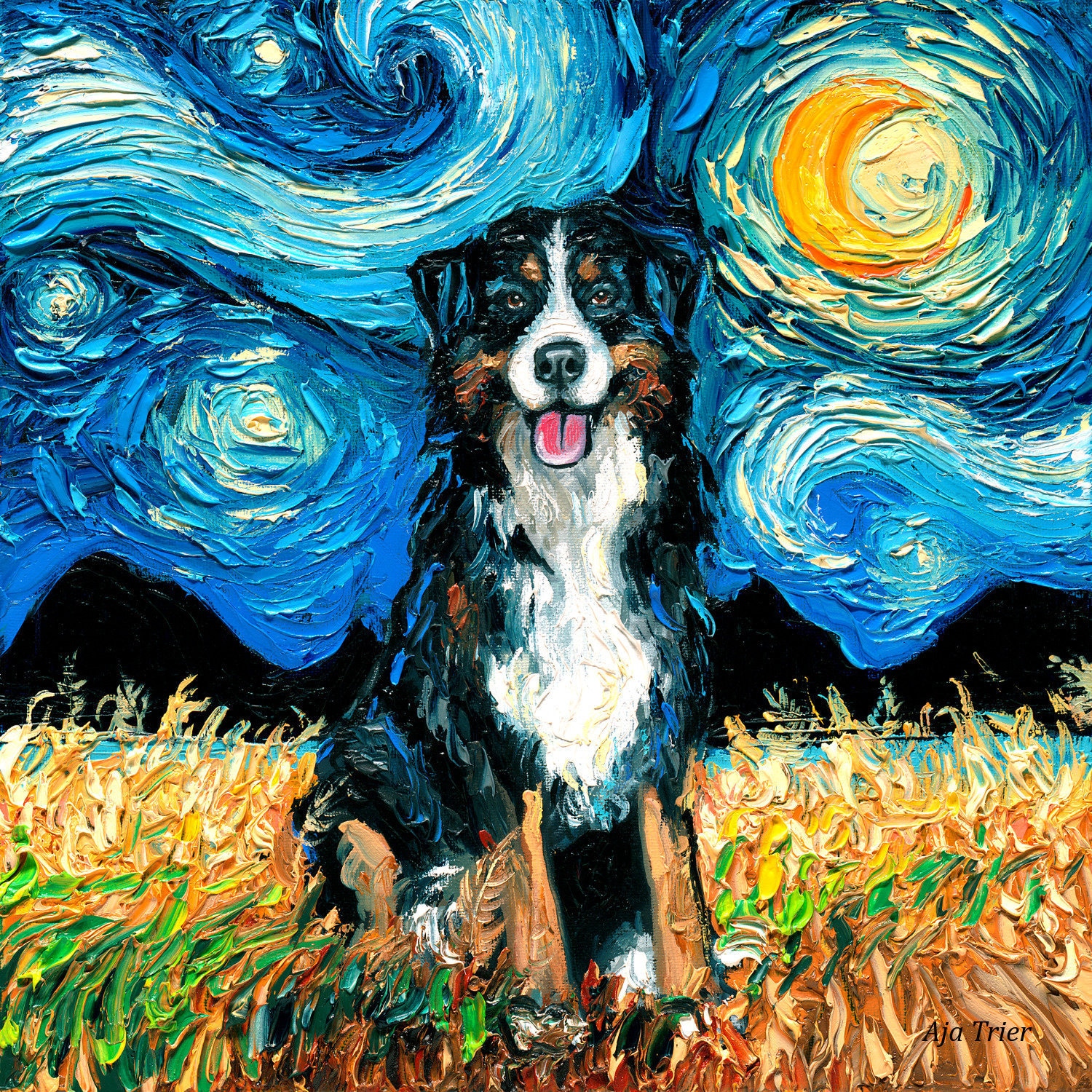This image is a square, portrait-oriented painting that creatively reinterprets Vincent van Gogh's "Starry Night." The upper part of the artwork features the signature swirling blue sky with a large yellow crescent moon situated in the right upper corner. Below the iconic sky, the landscape transitions into a dark area, eventually giving way to a mix of dried brown grass with some patches of green grass in the foreground.

Dominating the center of the painting is a Bernese Mountain Dog, sitting down with all four legs on the ground. The dog is depicted in a pose with its mouth slightly open and its tongue sticking out, exuding a friendly demeanor. Its fur is primarily black, accented with light brown highlights around its eyes, mouth, and legs. The nose area and chest are distinctly white, providing a sharp contrast to the rest of its body.

The entire painting emulates Van Gogh's chunky, textured brushstroke style, adding a vivid, textural quality to the scene. In the bottom right-hand corner, the artist's signature "AHA TRIER," rendered in black letters, completes the composition, merging classical inspiration with a whimsical canine centerpiece.